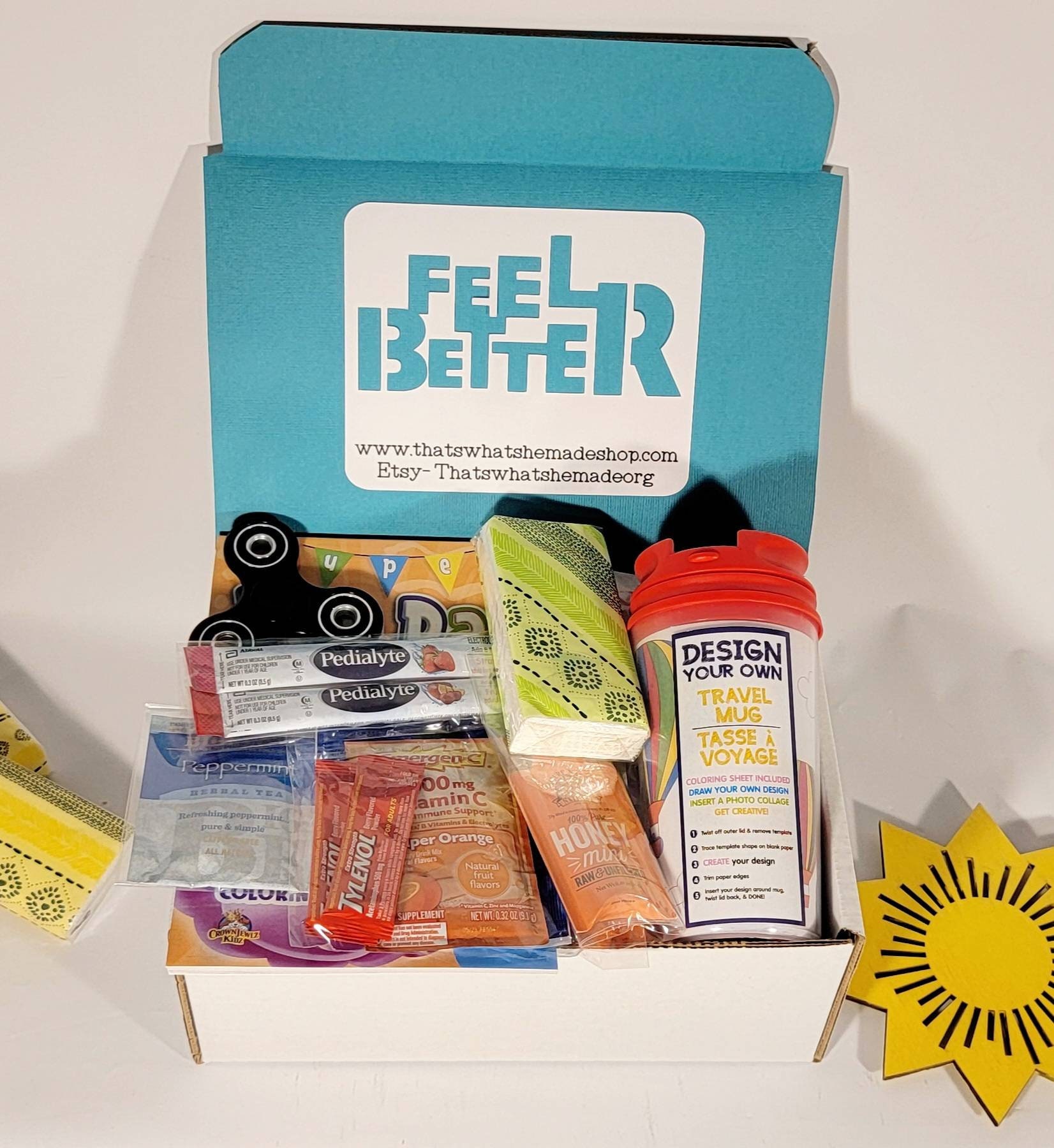The photograph captures a care package prominently placed on a white table. This thoughtful package features an open blue box with the message "Feel Better" in white lettering on the lid, accompanied by an Etsy shop address below. Inside, a variety of wellness essentials are neatly packed. Among the items are packets of Pedialyte, Tylenol, herbal peppermint tea, vitamin C, honey mint (labeled as 100% pure), a "design your own travel mug" kit, tissues or napkins, and possibly a fidget spinner. Surrounding the care package, the setting includes cheerful yellow decorations—a sun-like shape on the right and a geometric design on the left—enhancing the heartwarming presentation of the medical supplies meant to uplift someone's spirits.